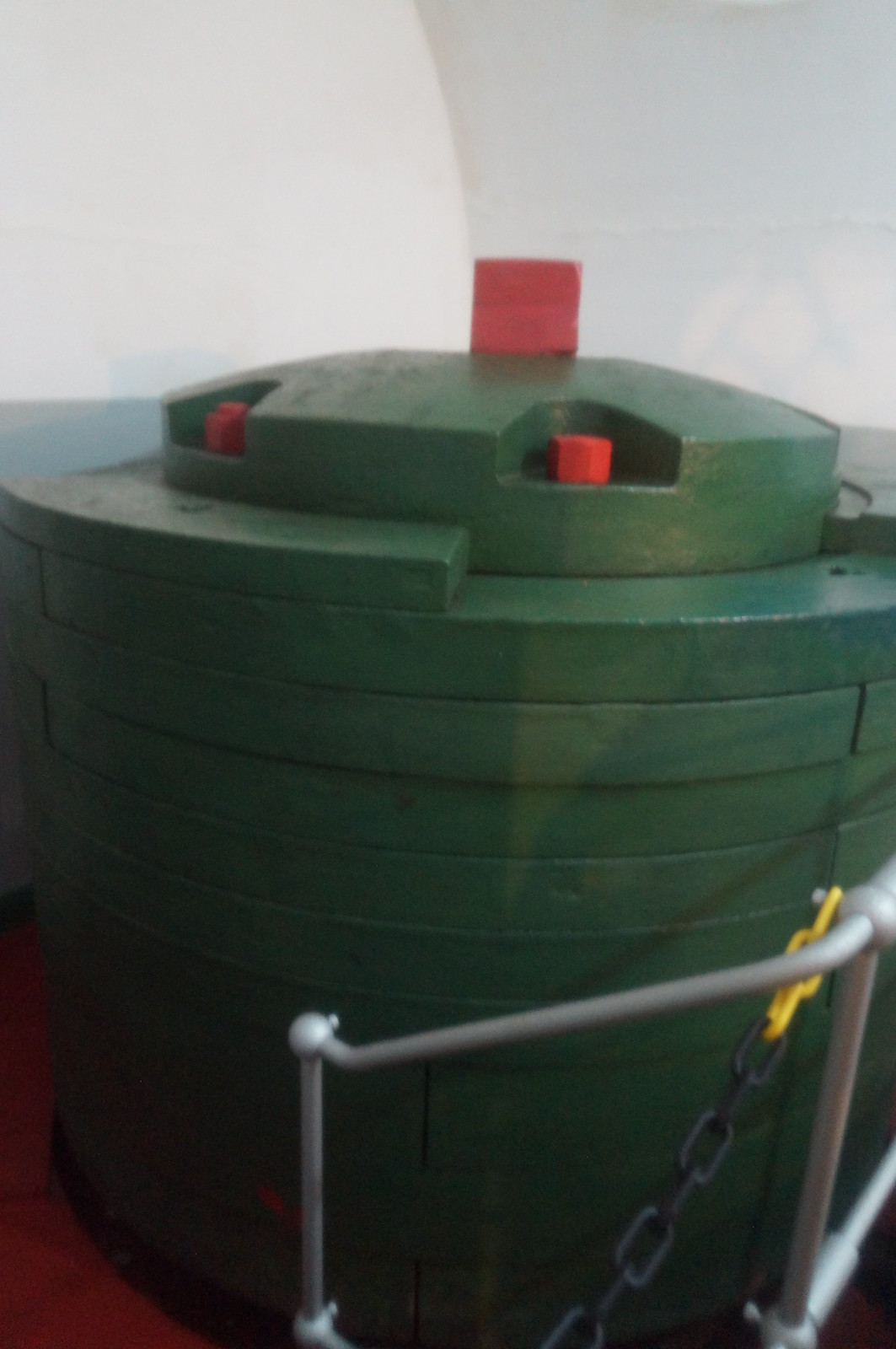The image is a color photograph in portrait orientation, showcasing a green cylindrical structure that appears to be either metallic or plastic. The camera is zoomed in tightly, so the left and right sides of the cylinder are cropped out of the frame. The cylinder is composed of stacked plates or concentric rings and is painted a dark green color. There are multiple red elements visible: a red surface near the bottom left corner on which the cylinder rests, and red pop-up tops—one smaller at the front and another larger at the back. Additionally, a red recessed area on the left side of the cylinder contains another red pop-up component. In front of this cylindrical structure, a gray metal fence is visible running from the right side towards the center. Attached to this fence is a chain with yellow and black links. The background features a white wall, adding contrast to the vibrant colors in the foreground.